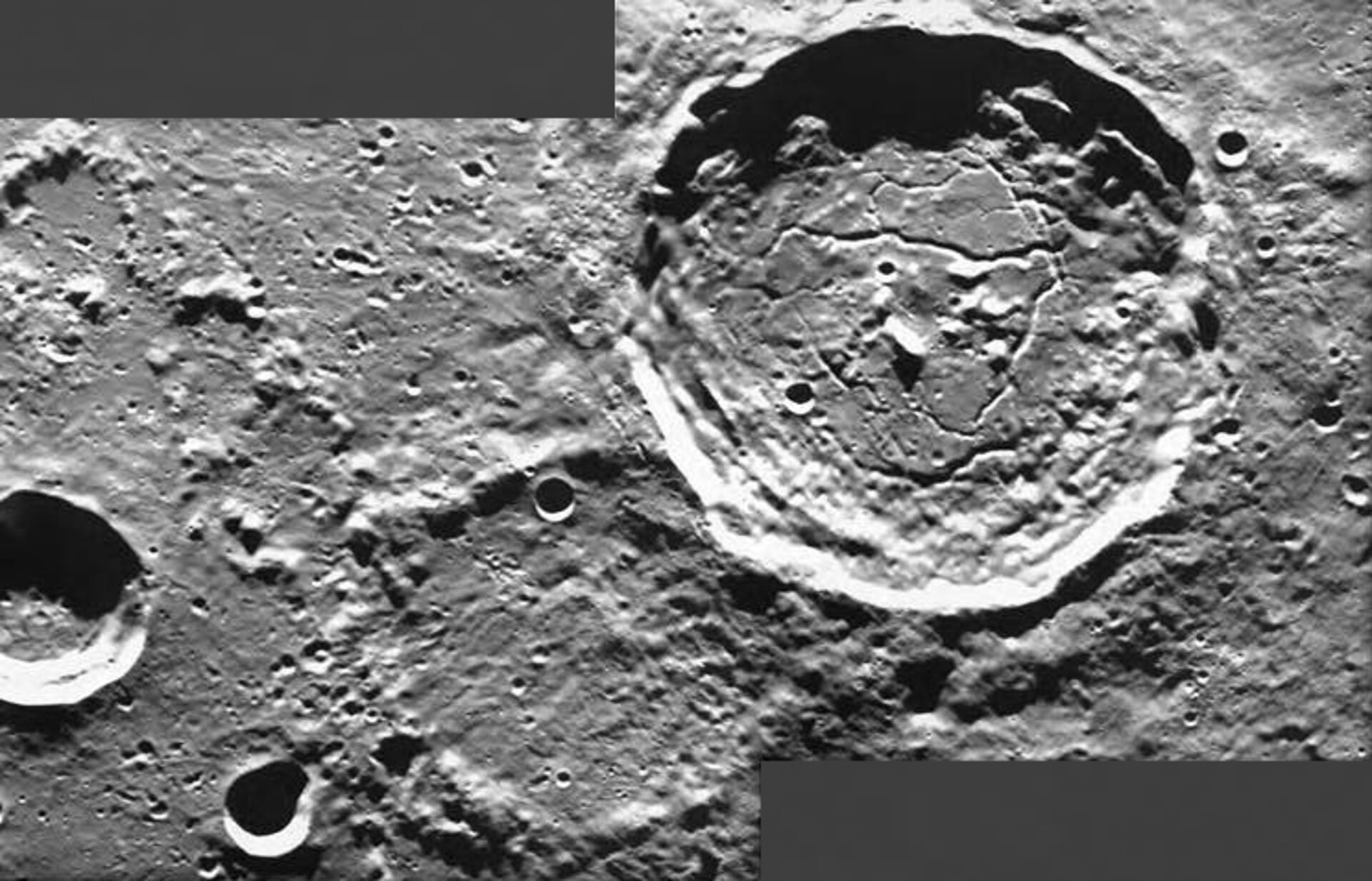This detailed grayscale photograph, captured through a telescope, features the rugged surface of the moon adorned with several impact craters of varying sizes. In the upper left, a notable gray rectangular mark frames the composition, while additional rectangular forms can be spotted in the bottom right. Prominent craters punctuate the lunar landscape, including one in the far left and another in the bottom left corner, as well as two large craters additional to these features. Subtle textures emphasize the moon’s jagged, craggy surface, dotted with small to large circular indentations characteristic of deep impact holes. The image provides an up-close view that emphasizes the varied and intricate details of the moon’s topography.